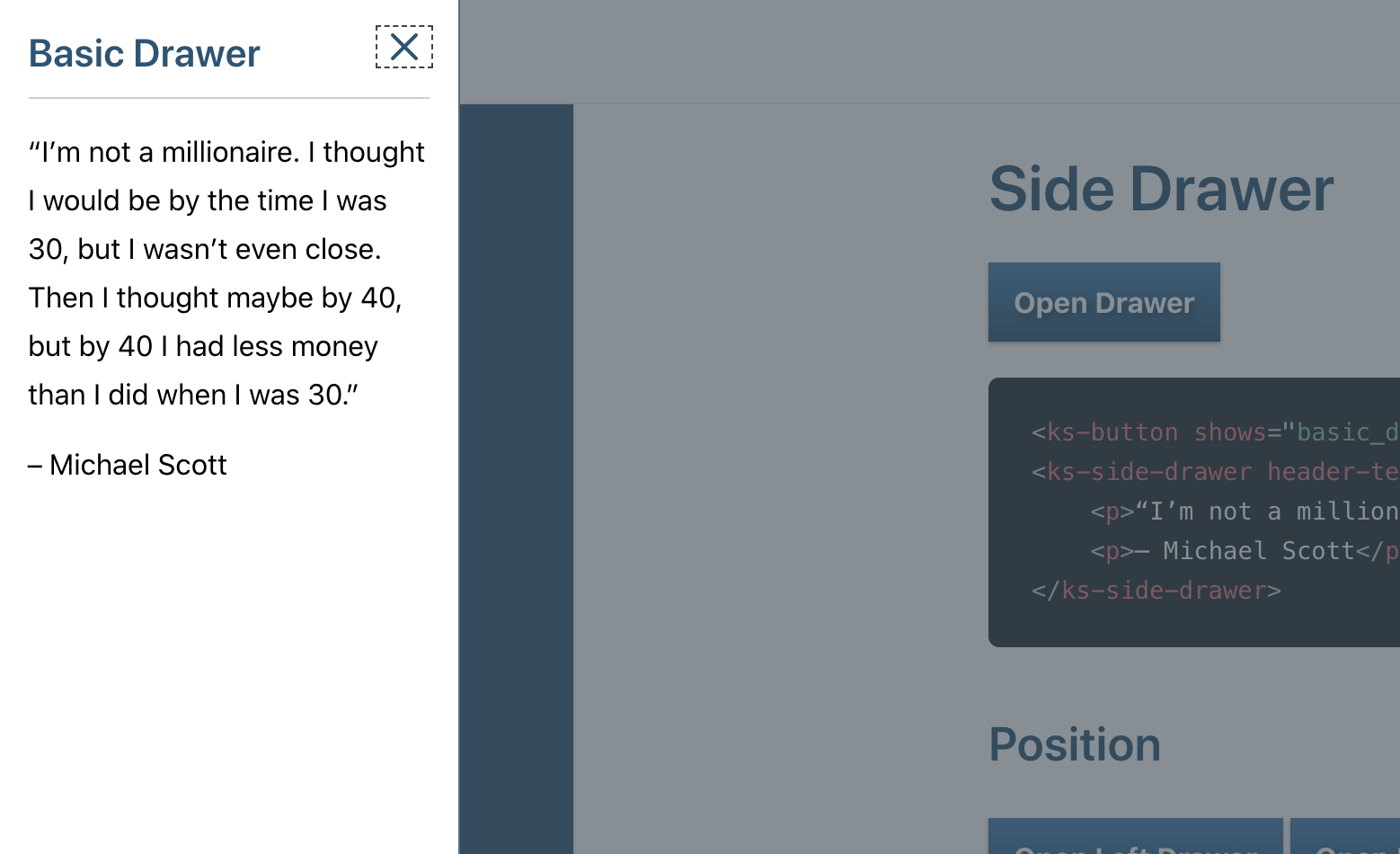The image features a series of labeled sections and text, beginning on the left side with the phrase "Basic Drawer" in blue text. Below this, there is an image of the letter "X" enclosed in a square. Further down, a quote reads, "I'm not a millionaire. I thought I would be by the time I was 30 but I wasn't even close. Then I thought maybe by 40 but by 40 I had less money than I did when I was 30," followed by a hyphen and the attribution "Michael Scott."

On the right side of the image, the only readable text begins with the label "Side Drawer," written twice, both times with the spelling "drawer" clarified as "d-r-a-w-e-r." Within a blue rectangle, the text "Open Drawer" appears in blue, followed by four lines of black text that are somewhat difficult to read: "KS-button," "KS-side drawer header," "side-drawer," and again "side-drawer." Exiting this box, the final piece of text in blue is the word "Position."